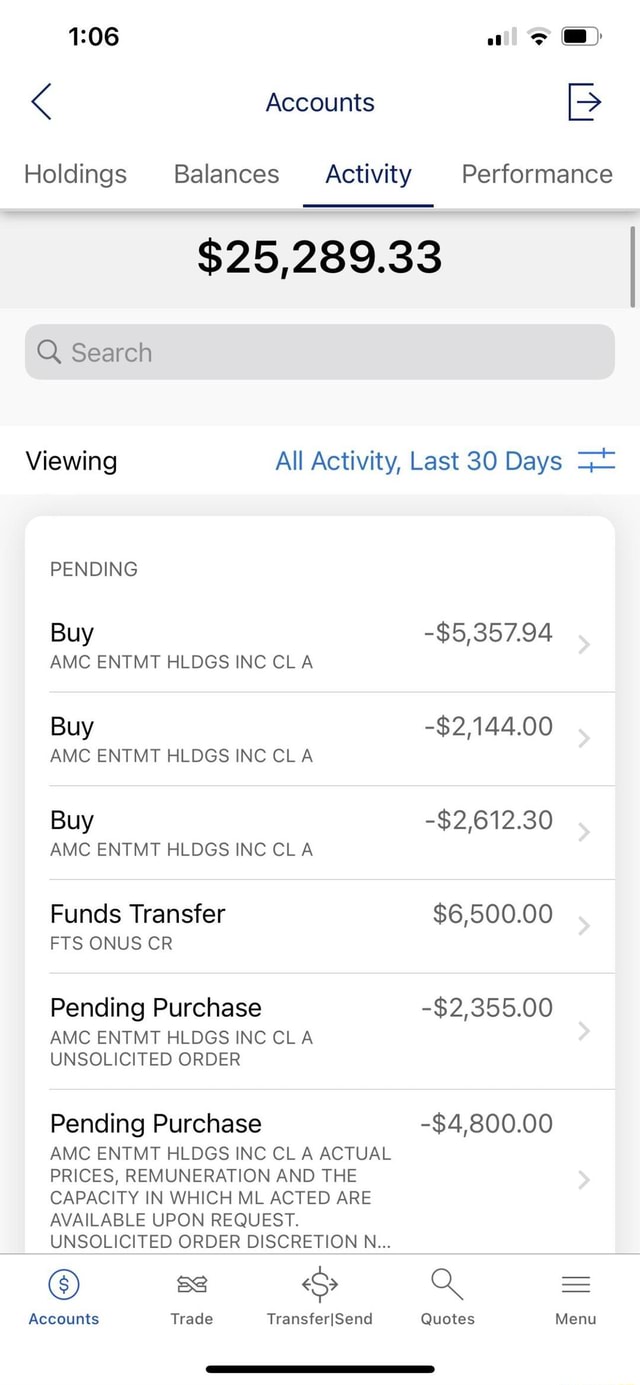Here is a detailed and cleaned-up caption for the provided image description:

---

The image depicts a screenshot of an account activity page. At the top of the screenshot, various status icons are visible, including the time, signal strength, Wi-Fi connection, and battery level indicators. Below these icons, the page title "Accounts" is prominently displayed, indicating that the user is within the account settings section of the app.

Navigating further down, the navigation menu is shown with options such as "Holdings," "Balances," and "Activity," with "Activity" being the currently selected and underlined tab. To the right, there is another tab labeled "Performance." Following this, a search bar is situated below the navigation menu, facilitating user searches within the activity feed.

The main body of the page specifies that the current view is "all activity in the last 30 days." The listed transactions are categorized and detailed as follows:
- Several instances labeled "Pending" and "Buy," each accompanied by respective amounts on the right.
- Multiple entries titled "Funds Transferred," also displaying amounts to the right.
- Entries noted as "Pending Purchase," characterized by longer detail descriptions alongside amounts on the right.

At the bottom of the screenshot, a menu bar provides quick navigation options with the labels "Accounts," "Trade," "Transfer," and "Send Codes" clearly visible.

---

This elaborated caption is structured and articulated to give a precise understanding of the screenshot's content while maintaining the necessary details.